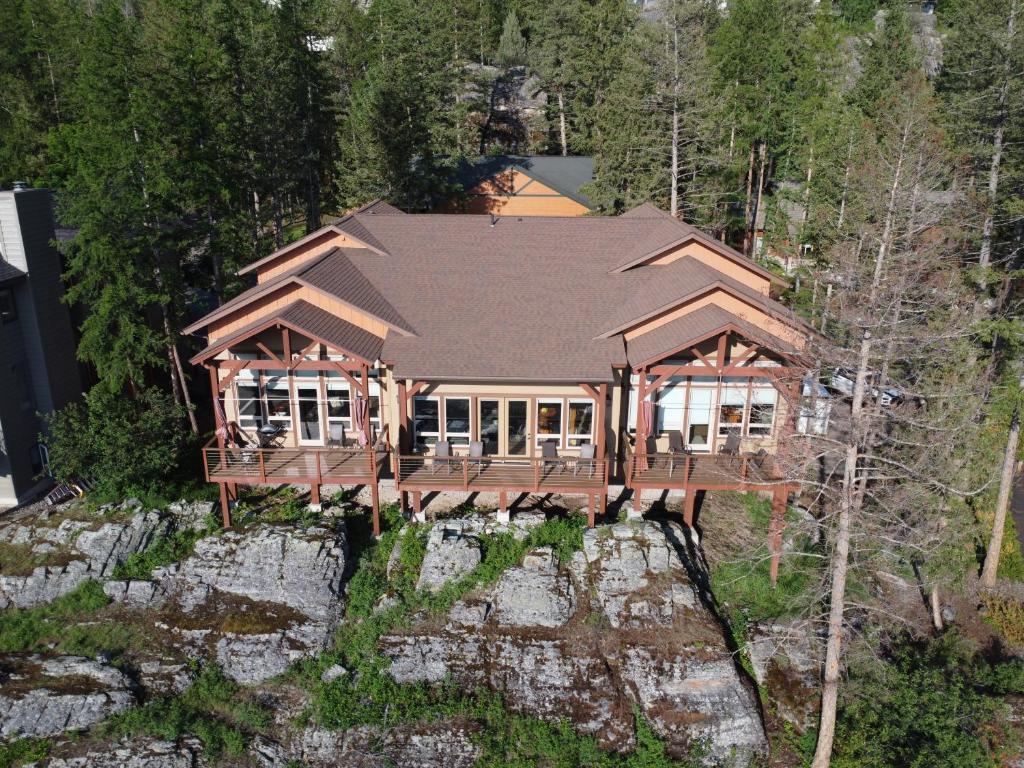This photograph showcases a large, multi-story house situated in the heart of a dense forest, captured from an elevated vantage point, possibly by a drone. The house is built on posts, lifting it above the rocky, partially vegetated ground. The structure features a wide deck in the foreground with numerous windows, and an exterior that combines white walls with brownish-orange and dark gray highlights. The roof sections visible include both typical dark gray and light orange components. 

The residence appears to be divided into multiple sections or units, possibly accommodating several families, given the separate entrances and individual decks. Each section of the house includes dark reddish-brown decks and a mix of white and brownish-trimmed windows and doors. There is a tree without leaves visible on the right side of the image, adding to the rugged, untouched ambiance of the surroundings. Patio furniture and a barbecue grill can be observed, suggesting the dwelling is well-equipped for outdoor living, despite its isolated location within the tall, green forest trees.